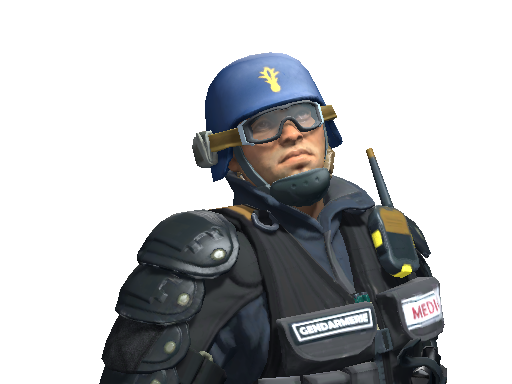This image portrays a video game-rendered depiction of a government police officer, possibly a SWAT team member or armored medic, seen from the chest up. The figure, resembling a white man with no facial hair, gazes slightly upward and slightly to the right. He is outfitted in detailed riot gear. Prominently featured is a blue helmet with a central yellow emblem resembling a sword with a radiating light pattern. Transparent goggles are attached to his helmet, with a chin strap and black chin protector securing it.

His upper body armor consists of a black vest worn over a dark blue jacket. The vest is adorned with several pouches, one at chest level with 'Medic' inscribed in white and another on the left side labeled 'Gend Armory.' A walkie-talkie is positioned above the left breast pocket. The vest's lower section houses a large utility belt, partially obscured. On his right arm, he sports protective padding with a series of three large pads extending from his shoulder down the arm, disappearing out of the frame.